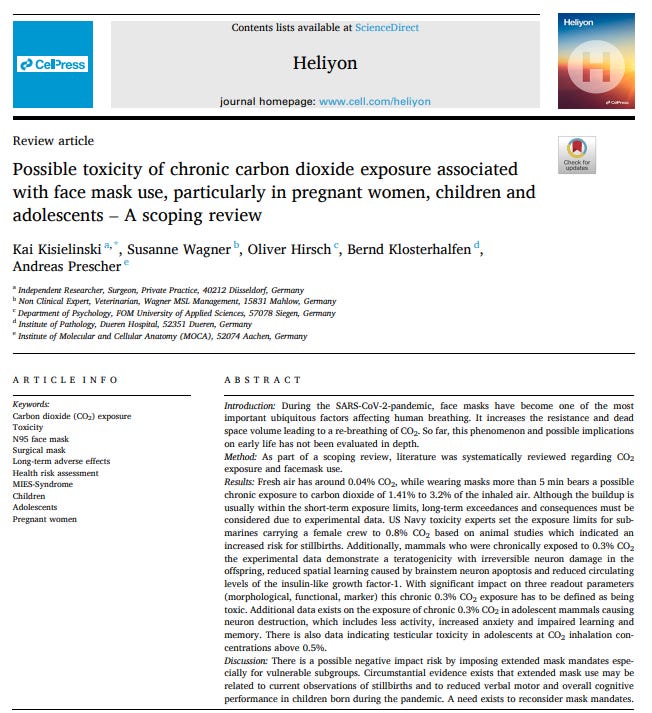This image depicts a webpage of a scientific article from the journal Helion, displayed on the Cell Press website. The top-left corner of the page features a blue box with the text "Cell Press," while the upper right corner shows a multicolored box labeled "Helion." Below, a note indicates that the contents list is available on ScienceDirect, and the journal’s homepage is provided at "www.cell.com/helion."

The article is categorized as a review piece and is entitled "Possible toxicity of chronic carbon dioxide exposure associated with face mask use, particularly in pregnant women, children, and adolescents: A scoping review." The authors listed are Kai Kisielinski, Suzanne Wagner, Oliver Hirsch, Bernd Klosterhäuflen, and Andrius Wischer.

On the left side of the page, there is a section labeled "Article Information," which includes a list of keywords: carbon dioxide exposure, toxicity, N95 face mask, surgical mask, long-term adverse effects, health risk assessment, MIES syndrome, children, adolescents, and pregnant women. The page also includes an abstract summarizing the article, although the specific content of the abstract is not visible in the image.